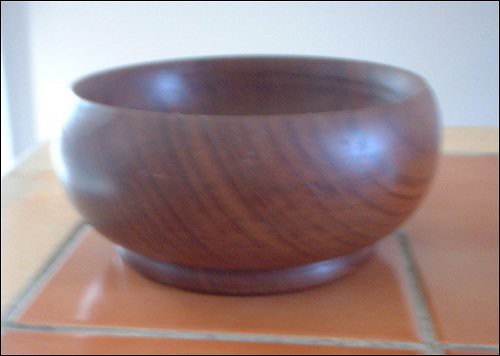In the image, we see a close-up of a darkly stained, wooden bowl sitting on a tile countertop, which could also be a table, reflecting light coming from the left. The bowl is not very large and features a distinct diagonal grain pattern that wraps around its circular shape, adding a textured design element. The wood's surface appears shiny, catching reflections of the ambient light. The tiles beneath the bowl are a dark brownish-orange color, bordered by grayish silver grout or caulk, giving the surface a defined structure. The countertop seems to have a border on the left side and at the top right corner. In the far background, a white wall adds contrast and depth to the scene, indicating that this setting is likely in a kitchen, possibly inside a home, though it could also be in a store. The overall image has a slightly blurry quality.